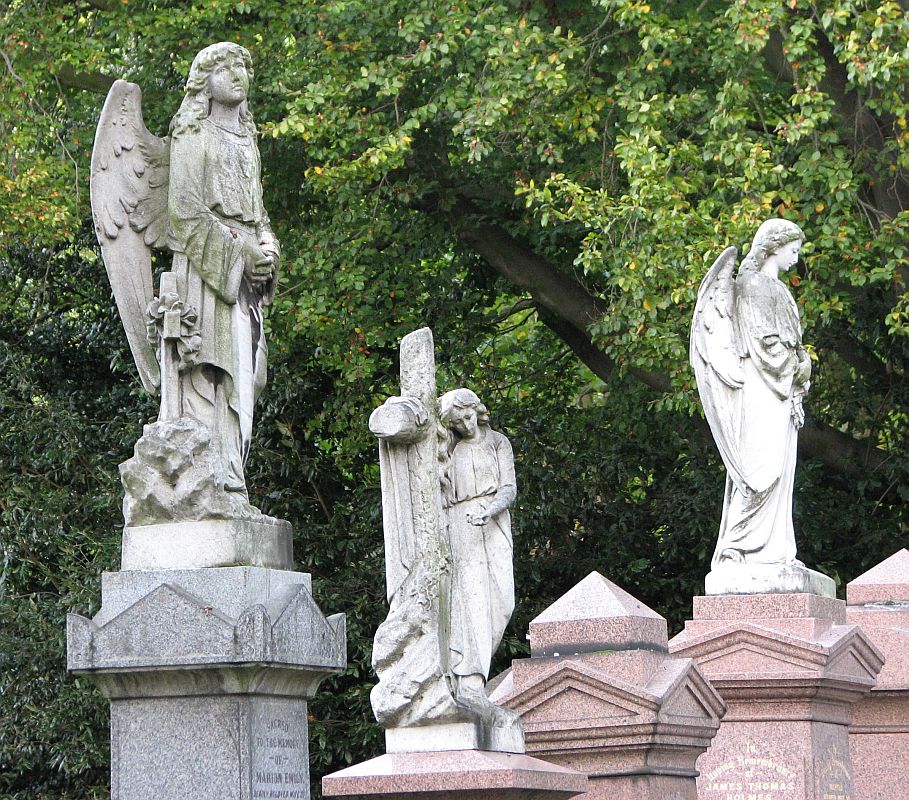This photograph captures an outdoor scene featuring a collection of aged, marble-like statues set against a backdrop of leafy tree canopies. There are three prominent statues: two angels and a woman. The angels, positioned on the left and right, each have majestic wings and flowing robes, conveying a sense of solemnity. The angel on the left looks upward with clasped hands, while the angel on the right stands tall and dignified.

In the center is a statue of a woman, perhaps one of the Marys from the biblical story of Jesus' crucifixion, as she leans her head against a wooden cross with a downcast and sullen expression. Her presence suggests mourning, possibly in the aftermath of Jesus' death. These sculptures, perched atop stone bases, evoke a somber narrative amidst the greenery of the surrounding trees, adding depth to the scene's melancholic atmosphere.